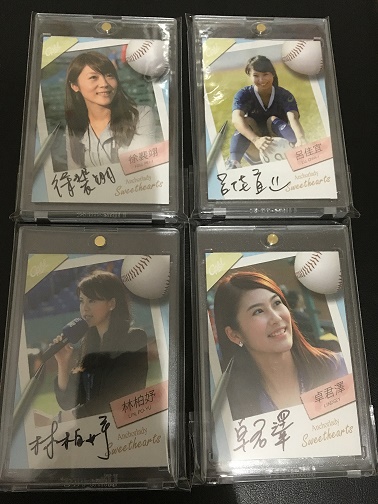This image captures a top-down view of four distinct baseball cards, each encased in clear plastic protectors. Each card features a unique photograph of an Asian girl, possibly Korean or Japanese, paired with various thematic elements, including a baseball in the upper right corner, a ribbon in the upper left corner, and a pin in the bottom left corner.

**Top Left Card**: This card showcases the girl with side bangs, looking to the right. Her image is in Polaroid-style, framed by a red ribbon on the left side, and features her autograph in the lower right corner.

**Top Right Card**: Here, the girl is depicted sitting on her knees, holding a soccer ball. This card includes her signature adorned with a smiley face.

**Bottom Left Card**: In this card, the girl is looking to the left, holding a microphone, and dressed in a suit. Her image maintains the same Polaroid-style format.

**Bottom Right Card**: The final card highlights the girl smiling brightly, showing her teeth, while looking to the right. Her facial expression conveys joy and enthusiasm.

Each card’s clear protective casing ensures the preservation of these detailed and vibrant images, combining personal memorabilia with artistic design elements.